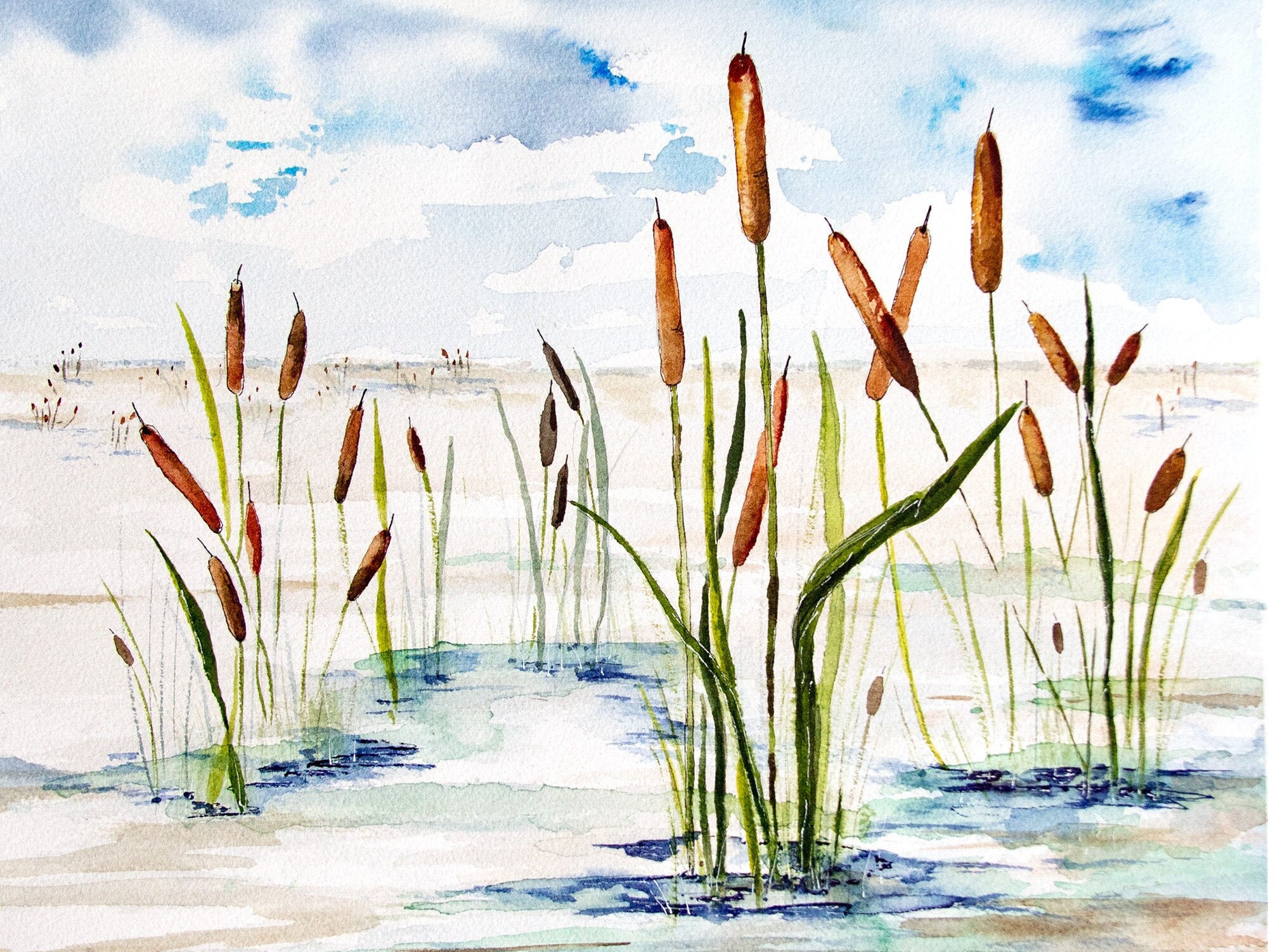This watercolor painting illustrates a tranquil swamp or marshland scene characterized by reeds emerging from the murky water. The water is partially covered by a cream to brownish foam, with dark blue patches breaking through at the bases of the reeds. The reeds are tall and slender with long, lime green leaves and feature large, oblong brown bulbs at their tips. In the foreground and background, these reeds dot the landscape, providing a rhythm to the scene. The sky above is partly cloudy, with deep blue tones peeking through the clouds, mirroring the dark blue water below. The overall composition of the painting, with its earthy browns and serene blues, creates a very calming and serene atmosphere, reflective of a natural, untouched swamp or marshland.